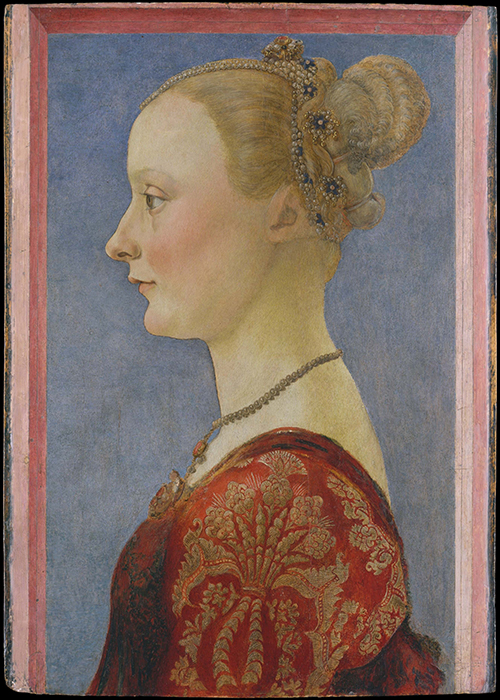This detailed and expertly rendered painting captures the left profile of a regal woman, likely of royal descent. The portrait is contained within a vertically arranged, rectangular frame featuring a light pink outer edge and a dark pink inner border. The background of the image is a serene light blue, adding depth to the composition.

The woman, depicted from just above her head to below her chest, exudes elegance with her meticulously styled blonde hair, which is swept up into an ornate bun or braid. Her hair is adorned with a gold and purple barrette, accessorized further with white and blue floral jewelry, reminiscent of headbands, enhancing her regal appearance. She has fair, almost white skin with a healthy blush or pink makeup on her cheeks. 

Her attire is equally splendid, boasting a rich ruby red garment adorned with intricate gold leaf-pattern designs. Around her neck, she wears a matching gold necklace featuring a striking ruby pendant that mirrors the color and opulence of her dress. The woman's expression is serene and thoughtful as she gazes off into the distance, her eye open and her lips gently closed.

The overall composition and fine details suggest the painting was created by a highly skilled professional, capturing not only the woman's royal bearing but also the rich textures and intricate patterns of her attire and adornments. The combination of colors and the expert use of light and shadow make this portrait a captivating work of art.